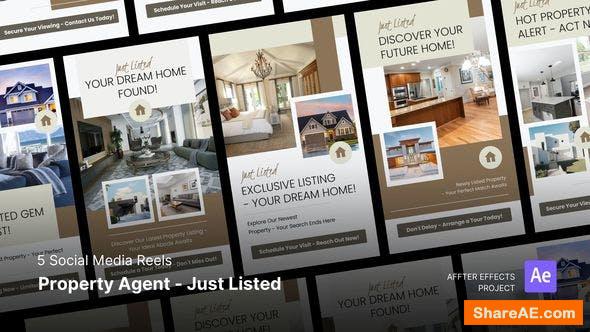The image appears to be a collage composed of various postings related to real estate. In the background, there are multiple snippets showcasing different homes, with phrases like "Just Listed," "Your Dream Home Found," "Exclusive Listing," and "Discover Your Future Home" visible among the images. These phrases are paired with corresponding pictures of houses, enhancing the visual appeal. 

On the bottom left of the collage, there's text indicating "Five Social Media Reels." Directly below this, in bold white letters, it reads "Property Agent Just Listed." Moving to the bottom right corner, the text "After Effects Project" is displayed. Adjacent to this, there's a small purple box carrying an uppercase 'A' and a lowercase 'e,' signifying the Adobe After Effects logo. Below this logo, in an orange button, it says "shareae.com," likely indicating the source or template provider for this project.

This collage appears to be an organized visual presentation intended for real estate marketing, utilizing a blend of eye-catching listings and promotional phrases to attract potential buyers.